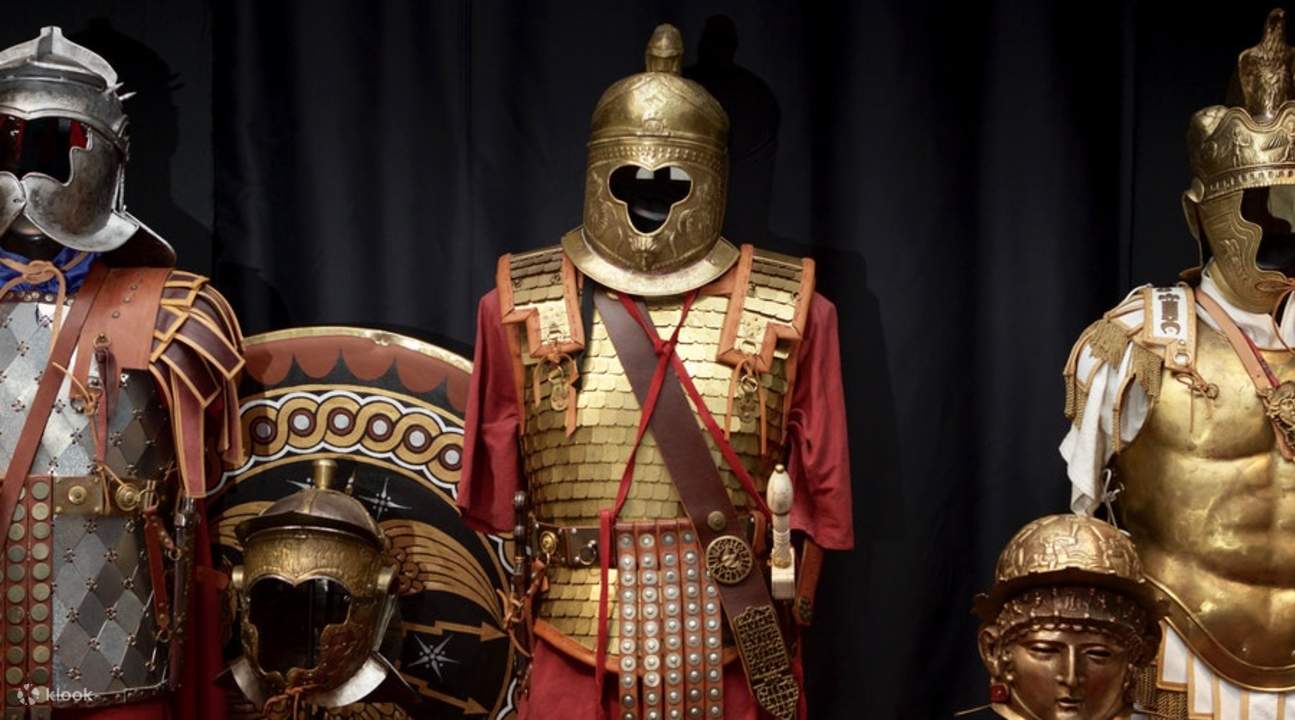The photograph showcases an elegant museum display of four suits of ancient Roman armor set against a black curtain backdrop. From left to right, the first figure stands adorned in a silver knight's outfit, complete with an open-faced helmet that covers the cheekbones and the lower nose. Immediately to the right, a silver helmet rests alone on a chair, juxtaposed with the figure who sits next to it, clad in a knight's outfit with a gold helmet and intricate details, including a red tunic, gold breastplate, and leather straps across his chest and sides, fastened with medallions. This figure also features a distinctive reddish tunic and a belt with five leather strips adorned with silver medallions. Further right stands another armor with a gold helmet and breastplate, distinguished by a white tunic and differing helmet design. Each armor, meticulously detailed, suggests the valor and artistry associated with Roman soldiers. Situated in the foreground, a golden youthful face mask adds to the intricate display, while a Roman shield with geometric designs subtly completes the scene in the background. This image vividly brings to life the grandeur and historical richness of ancient Roman armor.